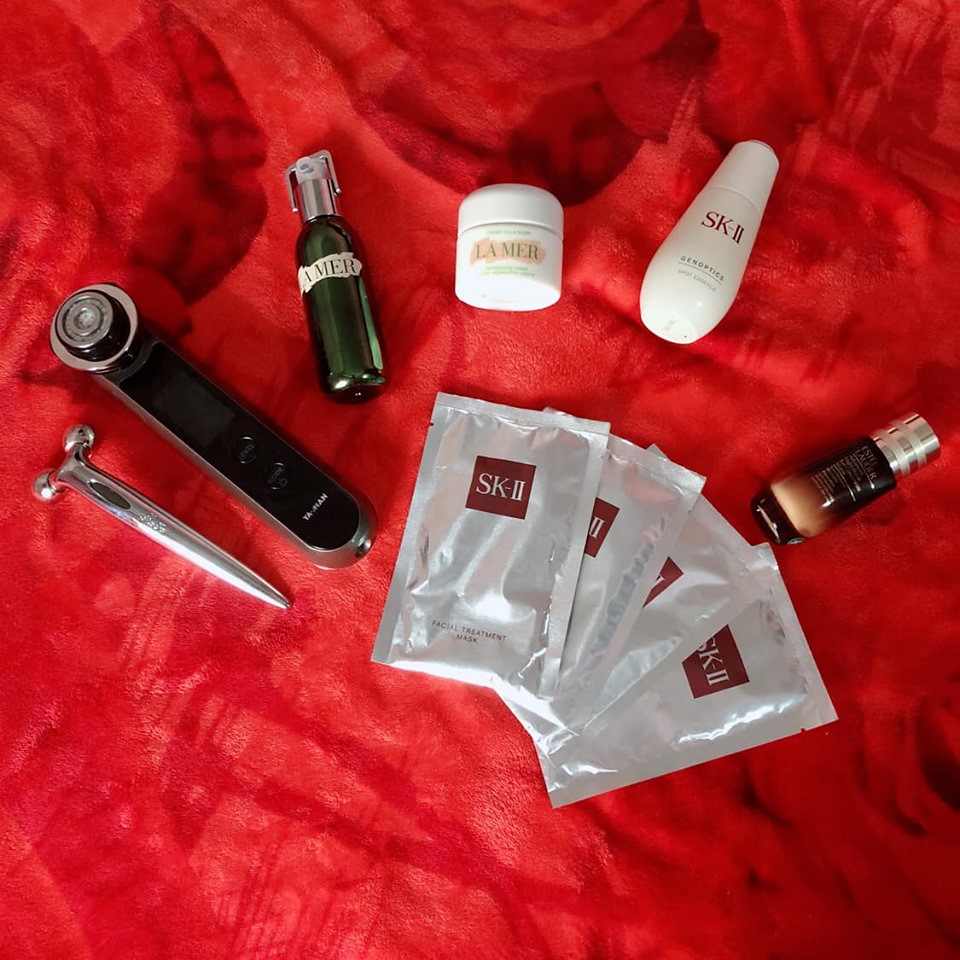This photograph showcases an array of high-end beauty products artistically arranged on a luxurious, red velvet fabric that boasts a rich texture with a distinct nap. Starting from the left, the first product is a sleek, silver facial roller, distinguished by its dual ball design at one end, used for facial massages. Adjacent to it is a sophisticated face shaver, characterized by its black body, adorned with black buttons, and a readable white label. The shaver features a circular head and is likely a versatile wet and dry option.

Next in line is an elegant, iridescent green bottle with a spray top capped by a silver lid. It sports a white label with bold black letters spelling "AMER" across the front. Following this is a refined, small white tub, embellished with a pink label featuring gold lettering that spells "LA MER." The tub also displays additional green text on its lower white portion.

To its right stands a pristine white bottle branded with red "SK-II" letters and accompanying black text. The subsequent item is a rich, gradient brown bottle, transitioning from a light tan at the bottom to a deep, dark brown at the top, capped with a chrome-finished lid accentuated by dual matte chrome bands. The bottle is adorned with gold inscriptions, adding a touch of elegance, although the text is not clear.

Positioned prominently in front of these products are four silver foil packets. Each packet features a red label presenting "SK-II" in silver letters, with "Facial Treatment Mask" inscribed in black at the bottom. The overall setup exudes a sense of luxury and sophistication, highlighting the premium nature of the beauty products.